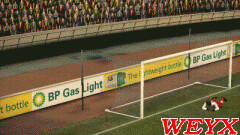In this pixelated video game screenshot, the scene is set in a soccer field with distinct details visible despite the game’s pixelation. At the top, extending from about 2 inches from the left to roughly an inch from the right and slightly angled upwards, is a crowd of indistinguishable spectators. Below the spectators, a concrete barrier runs in front of them, accompanied by a fence that stretches across the view. Descending further, there's a green wall followed by a small gray strip, and below this strip, a dirt patch angling upward from left to right.

A long banner, angled similarly, follows; it features a yellow section with unidentified green lettering and a white section with green text reading “BP Gas Light.” Another dirt patch lies below the banner. In the foreground on green grass, there is a soccer goal with a white frame. A person in a white shirt and red pants, additionally sporting a black hat and black shoes, is lying on the ground in front of this goal. Prominently displayed in the bottom right corner of the image are the letters “W-E-Y-X” in bold red font. The overall scene, capturing the essence of a soccer match environment, is rendered in a style typical of vintage video games.